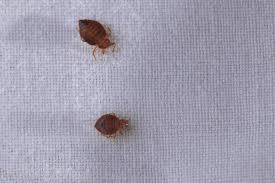The close-up image showcases a detailed view of two bed bugs on a white fabric, likely a sheet or blanket. The fabric's tight weave is clearly visible, revealing the intricate thread patterns. The bed bugs exhibit a red-brown coloration with rounded, flat bodies that have a somewhat leaf-like shape, ending in a sharp protrusion. The top bed bug, larger than the other, is positioned with its tail towards the top of the image and head angled to the bottom right. The smaller bed bug is located about three-quarters of an inch below, oriented with its tail to the left and head to the right. A faint, dark trail follows their path across the fabric, possibly a shadow or residue. The bed bugs appear dead and meticulously arranged for the photograph, likely evidencing an infestation.